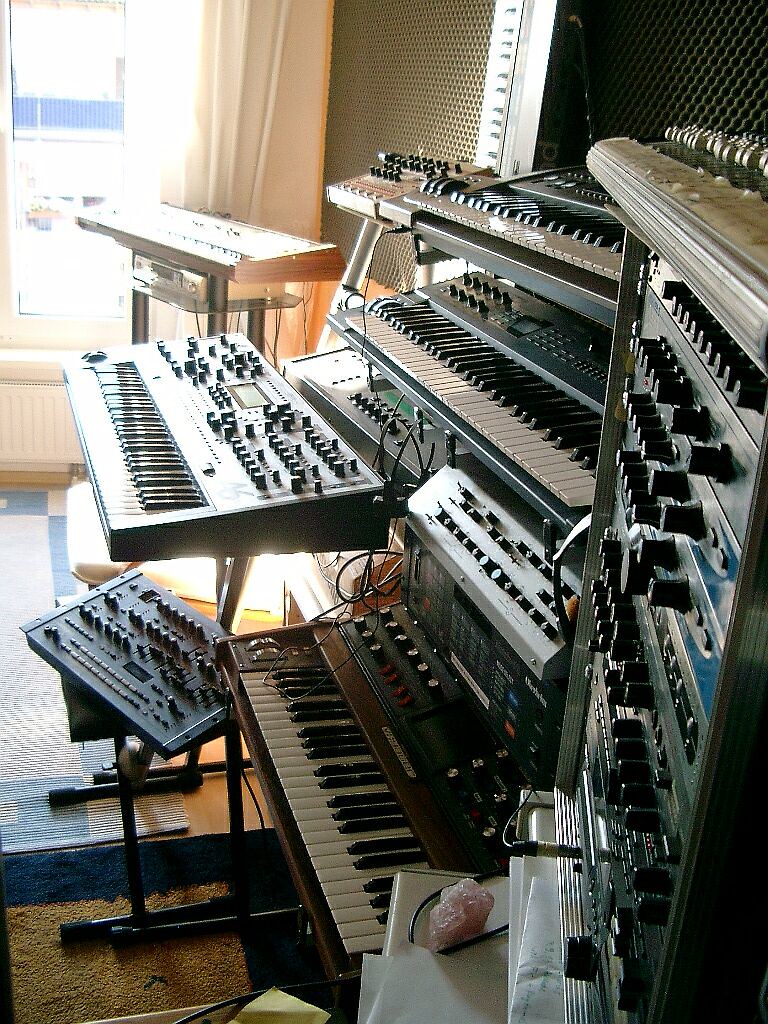The picture captures a bustling music room bathed in daylight from an open window or door in the far left-hand corner, revealing the partial view of another building outside. The room features a hardwood floor adorned with multiple area rugs and tapestries. Towards the right-hand side and throughout the room, an impressive array of musical instruments and equipment is visible. Numerous keyboards of different sizes and colors, mainly featuring black and white keys, are strategically placed; some are stacked on stands while others rest on flat surfaces. The space is packed with various tuning equipment, equalizers, dials, jacks, inputs, amplifiers, and speakers, indicating a well-equipped studio setup. Curtains or tapestries hang in the corners, adding to the room's creative ambiance. This intricate arrangement of musical gear, all facing away from the photographer positioned in the far right corner, showcases a dedicated music production environment.